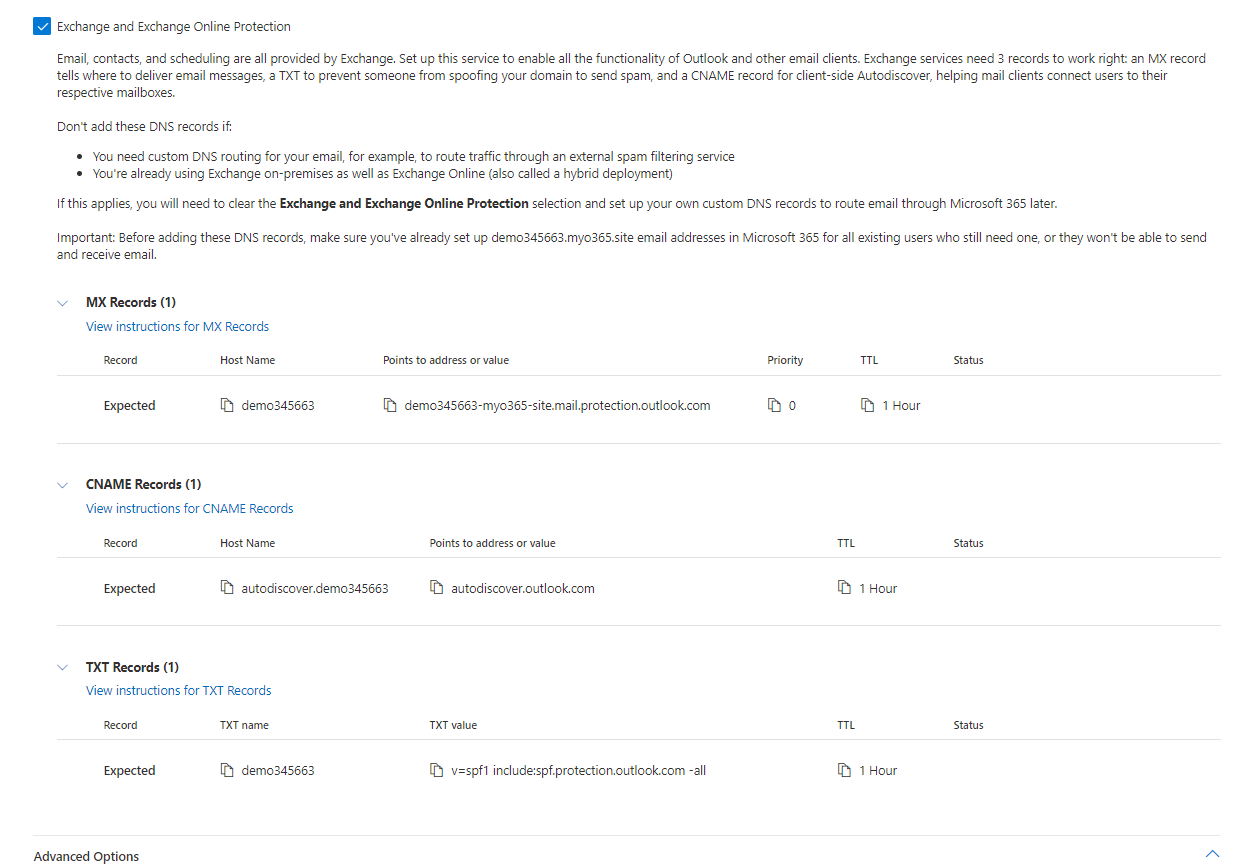**Screenshot from a Website Detailing Exchange and Exchange Online Protection Settings**

The image showcases a clean, white background with detailed instructions about setting up Exchange and Exchange Online Protection. At the top, a small blue square with a white checkmark inside is prominently displayed. Adjacent to the icon, in black text, are the words "Exchange and Exchange Online Protection."

Below this header, a description explains:
- “Email, Contacts, and Scheduling are all provided by Exchange. Set up this service to enable all the functionality of Outlook and other email clients.”
- “Exchange services need three records to work correctly: an MX record, a TXT record, and a CNAME record.”

The description further elaborates:
- **MX Record**: Instructs where to deliver email messages.
- **TXT Record**: Prevents domain spoofing for sending spam.
- **CNAME Record**: Facilitates client-side auto-discover, helping mail clients connect users to their respective mailboxes.

An important note is highlighted:
- “Do not add these DNS records if you need custom DNS routing for your email. If you have already signed up using both Exchange on-premises and Exchange Online, you will need to clear the Exchange and Exchange Online Protection settings.”

Following the descriptive guidelines, it provides specific details on:
- **MX Records**
- **CNAME Records**
- **TXT Records**

For each type of record, the image lists:
- Host Name
- Points to Address Value
- TXT Value
- TXT Names
- Priority
- TTL (Time to Live)
- Status

This detailed screenshot acts as a comprehensive guide for setting up and understanding the necessary DNS records for Exchange and Exchange Online Protection.